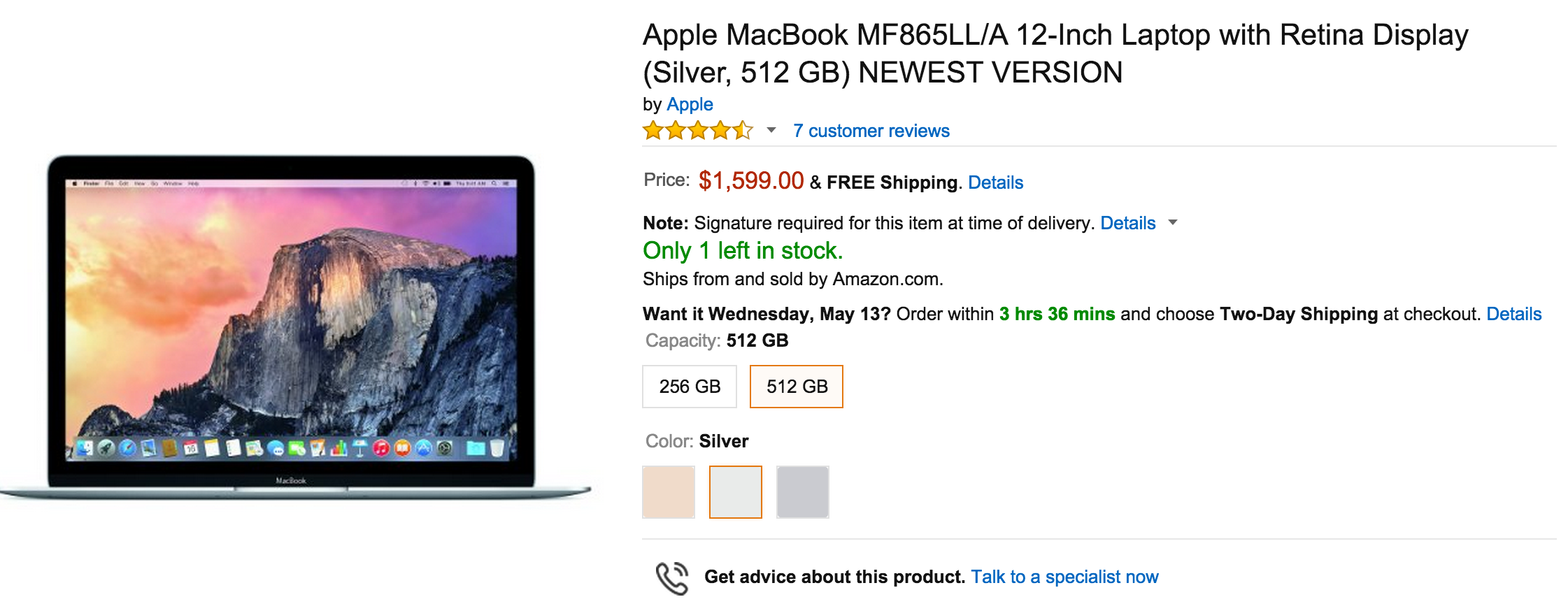The image showcases an Amazon shopping page displayed on a sleek Apple MacBook laptop. The laptop is set against a pristine white background, drawing attention to its glossy silver finish and elegant design. On the laptop's screen, a breathtaking mountain landscape is visible, with a prominent large peak accompanied by smaller ridges. The sky transitions from a violet hue at the top to a warm orange near the horizon, dotted with soft clouds.

At the top of the screen, a menu bar is present, while the bottom features various application icons, indicating the use of either macOS or Safari. The right side of the screen highlights detailed product information: it's an Apple MacBook model MF865LL4-A. This particular model is a 12-inch laptop boasting a Retina display, available in silver, with 512 gigabytes of storage. It is noted as the newest version and has garnered a rating of four and a half stars from seven customer reviews. The price is prominently displayed in red as $1,599 with the added benefit of free shipping. The text alerts potential buyers that only one unit is left in stock. Below the price, options for different storage capacities (512 GB and 250 GB) and color variations are available.